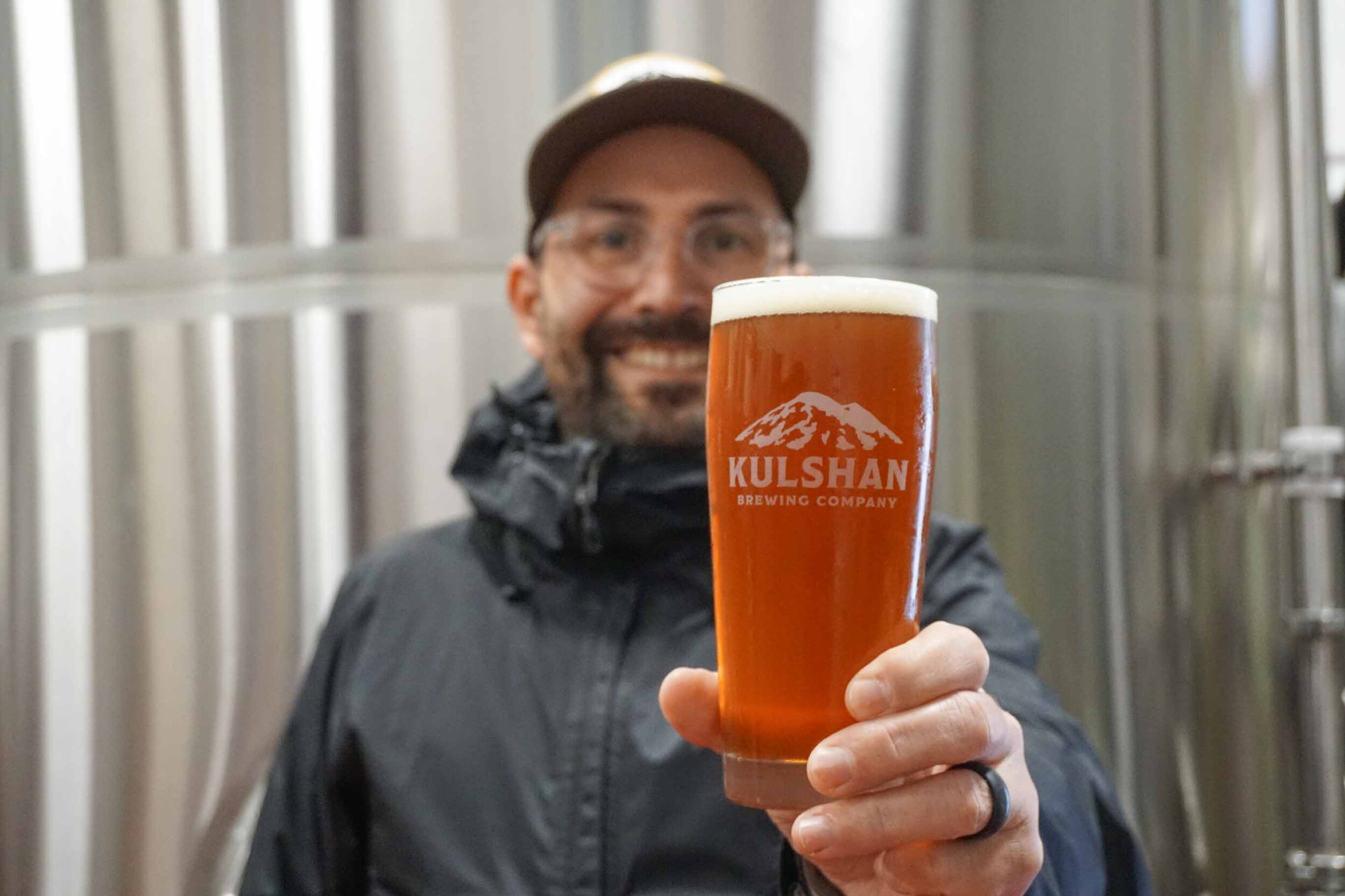In this advertisement photo for Cool Sean Brewing Company, a smiling man proudly holds a glass of freshly poured, deep amber beer, potentially a red ale. The company's logo, which features "Kulshan Brewing Company" in white text beneath an illustration of mountains, is prominently displayed on the glass. The man is slightly out of focus, as he holds the beer forward toward the camera. He has a full beard and wears clear-framed glasses, a black windbreaker with a hood, a baseball cap, and a black wedding ring. Behind him, silver brewing tanks can be seen, adding to the authentic brewery atmosphere.